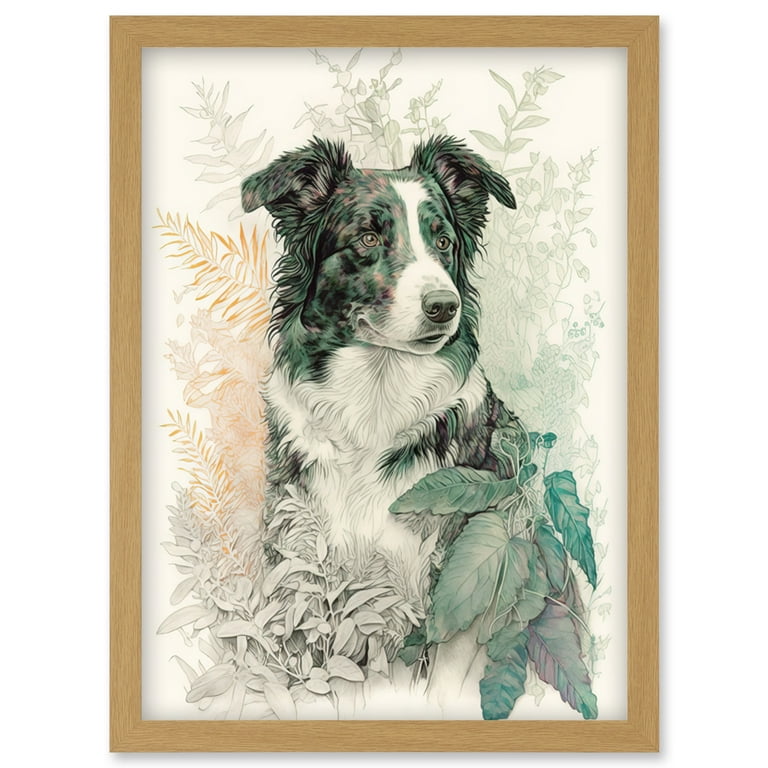This framed artwork showcases a detailed drawing of a dog, prominently displayed within a thin, light-colored wooden frame that measures a subtle shade of light brown. The composition features the dog surrounded by an intricate array of foliage, visible from the chest up. The foreground is adorned with a variety of leaves, including vibrant green and muted gray ones. In the background, autumnal orange leaves and a pale, light green leaf provide additional layers of depth and color contrast.

The dog, rendered with meticulous attention to detail, boasts predominantly black fur, interspersed with subtle hints of red that add richness to its coat. Its face is marked by a striking white nose and a distinctive white stripe that runs between its eyes, broadening slightly at the forehead. This white marking extends to its neck and belly, providing a stark contrast to the predominantly black fur. The detailed rendering captures the essence of the dog's features and the play of light and shadow, emphasizing the artist's skill and attention to detail.